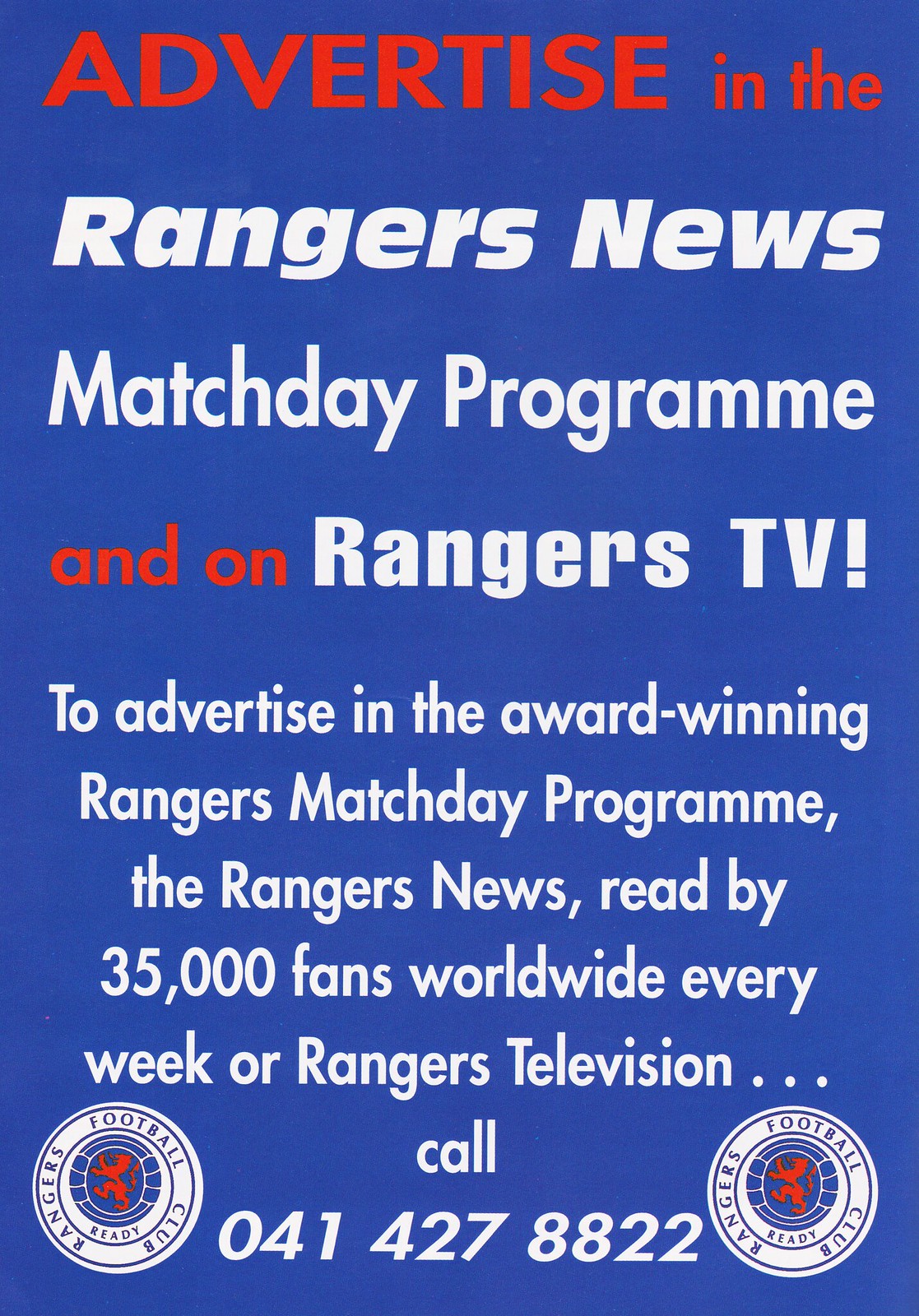The image is a vertically-oriented advertisement or flyer with a solid dark blue background and an intricate layout of text and graphics. At the top, in prominent red text, it reads, "Advertise in the", followed by white text stating, "Rangers News Match Day Program and on Rangers TV." The phrase "and on" also appears in red text. The body of the flyer contains white text encouraging interested parties to advertise in the award-winning Rangers Match Day Program. It reads: "To advertise in the award-winning Rangers Match Day Program, the Rangers News read by 35,000 fans worldwide every week, for Rangers Television, call 041-427-8822."

The bottom corners feature a repeating circular emblem with a white circle bordered in blue, containing the blue text "Rangers Football Club." At the center of the flyer, there is an artistic depiction of a soccer ball emblazoned with the image of a lion, creating a striking visual focus in the advertisement.